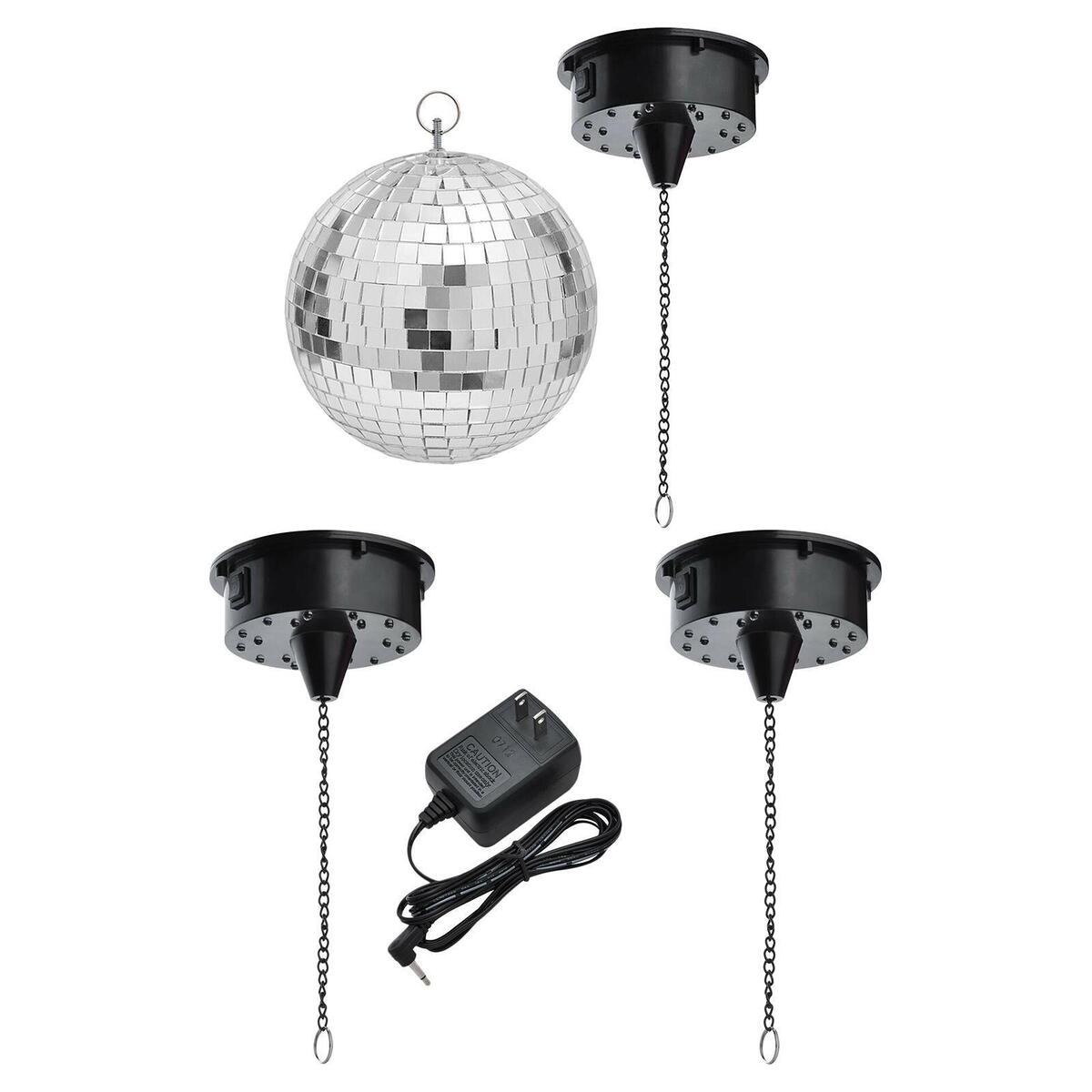In the image, there's a detailed setup for a hanging disco ball, perfect for a party atmosphere. Central to the scene are three black motorized pucks, each equipped with a switch on their left side and a plug-in port, likely designed for either 9-volt or 5-volt power sources. From each puck descends a silver chain, forming a cradle for the single disco ball with its typical shiny square mirrors. This ball hangs from a central chain, attached securely to one of the pucks. The setup suggests that the pucks not only provide structural support but also potentially light up and spin the disco ball when powered, adding dynamic lighting effects. The components, made of both plastic and metal, appear to include various parts that possibly connect to the ceiling and to a power source, ensuring the entire assembly operates smoothly to create a lively party environment.